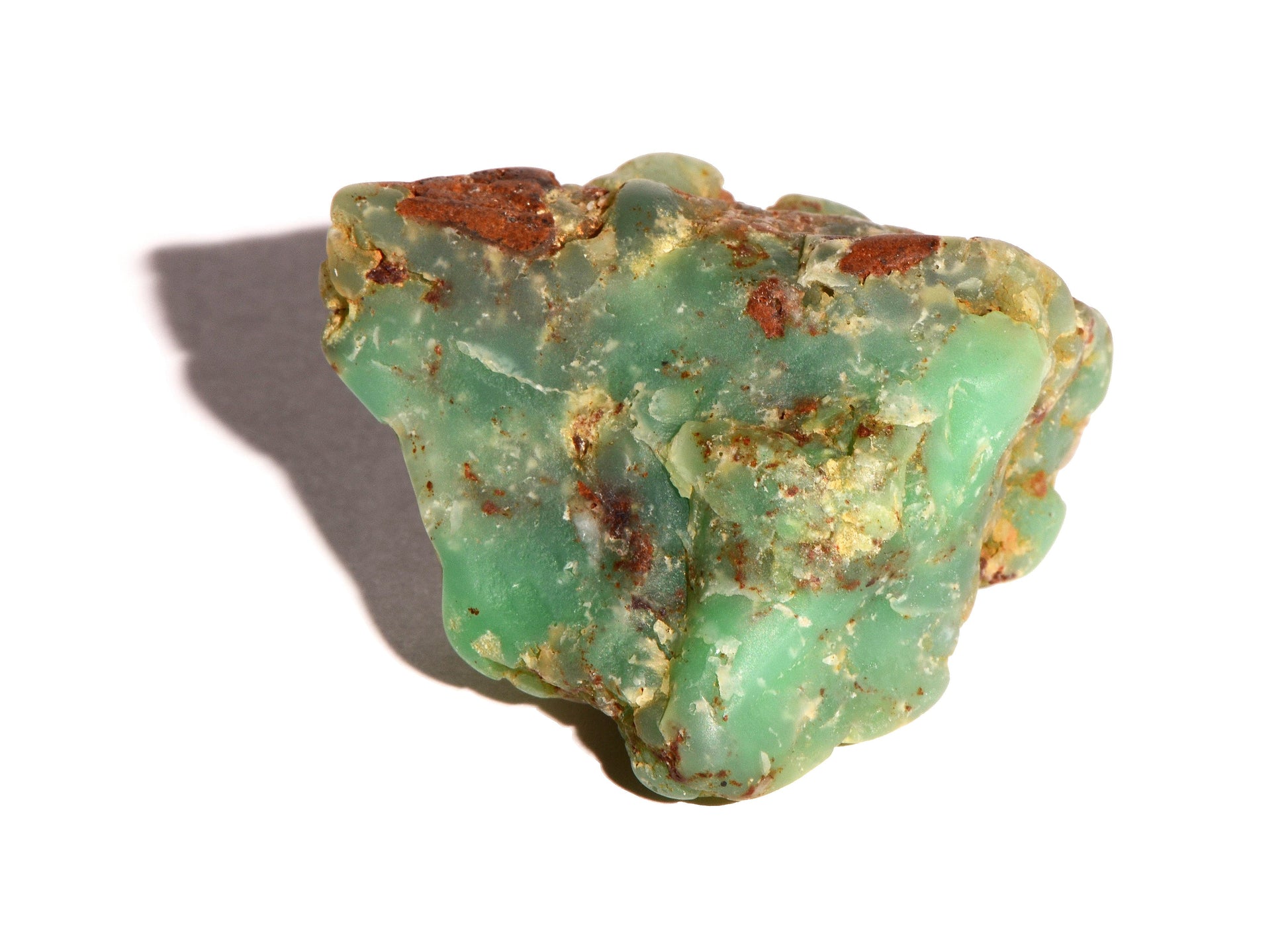The image showcases a striking mineral block, predominantly green, formed by a chemical reaction between a metallic substance and sulfur, likely copper sulfate or perhaps iron sulfate. This medium-sized, asymmetrically shaped block features elements of rust orange streaked throughout, with additional spots of yellow and gray. The rock-like mineral has an uneven surface, appearing lumpy with several small cracks. Its vivid coloration—a mix of turquoise, cyan, and green—adds to its intriguing appearance, while a shadow cast in the background reveals no other objects, emphasizing the mineral's distinct form and speckled textures.